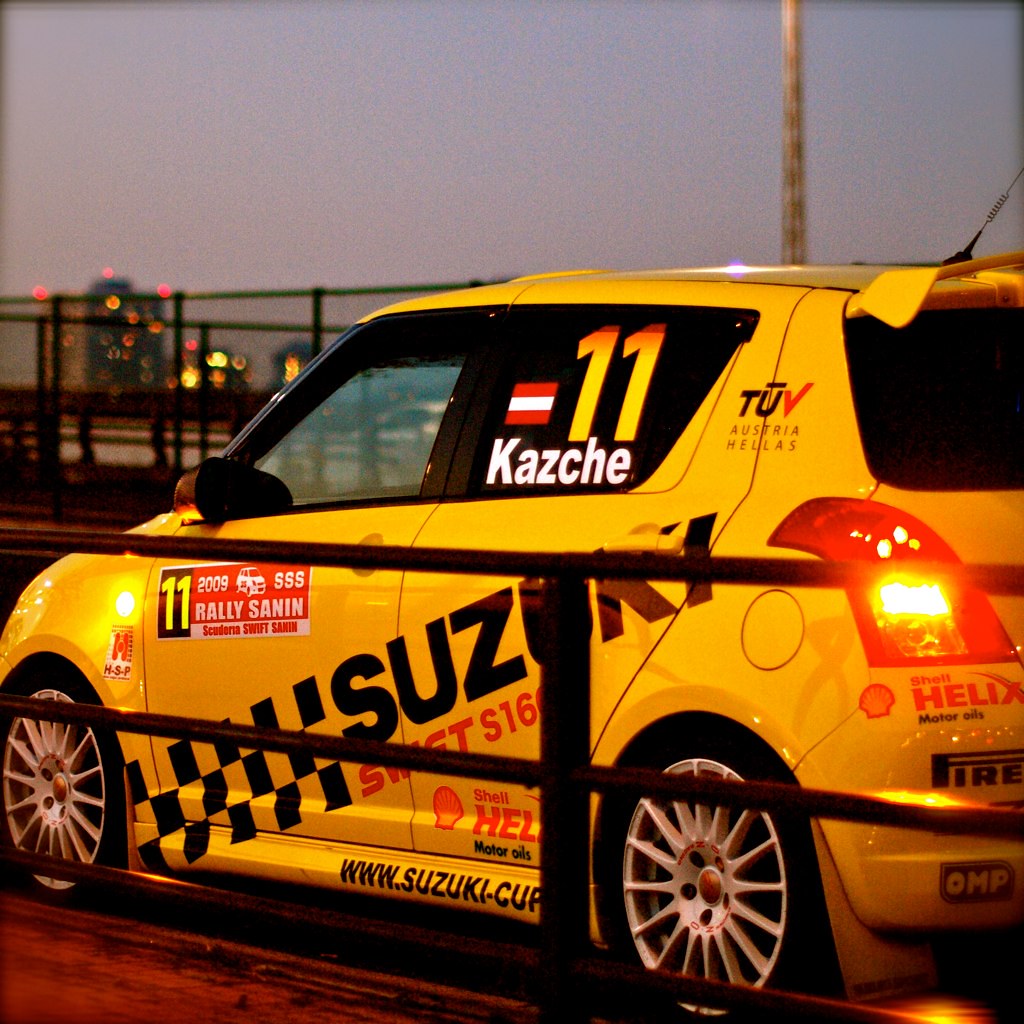The image depicts a vibrant yellow Suzuki subcompact rally car illuminated under the fading light of dusk, with a backdrop of distant skyscrapers and fencing. The car, striking and meticulously detailed, features black and bold Suzuki branding on its side and sports the number 11 displayed prominently on a black background. Adorned with a variety of graphics and advertisements including Pirelli, Shell, and a web address www.suzuki-cup, the vehicle conveys its racing pedigree. A notable detail is the red-white-red striped horizontal flag bearing the name Kazchei, marking its participation in the 2009 Rally Sunning event. It also boasts white wheels, a rear wing, and visible rear taillights, signaling its ready-for-action stance amidst the serene setting.